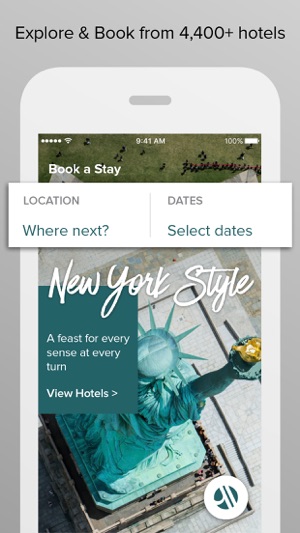The screenshot features a website with a lavender-colored background and prominent, bold black text that reads, “Explore and book from 4,400+ hotels.” Below this text, there is an illustration of a pale lavender cell phone, with most of the device visible except for the bottom of the screen. 

On the cell phone’s display, we see an aerial color image of the Statue of Liberty, showcasing the statue's grayish-silver hue and her iconic raised flame. The flame is highlighted by white text that reads “New York style.” Additionally, below the image is a blue box with white text proclaiming, “A feast for every sense at every turn,” followed by a “View hotels” call-to-action button. 

Towards the lower section of the screenshot, there are input fields for users to enter their travel details. The location field is labeled “Where’s next?” and there is a date field labeled “Select dates.”